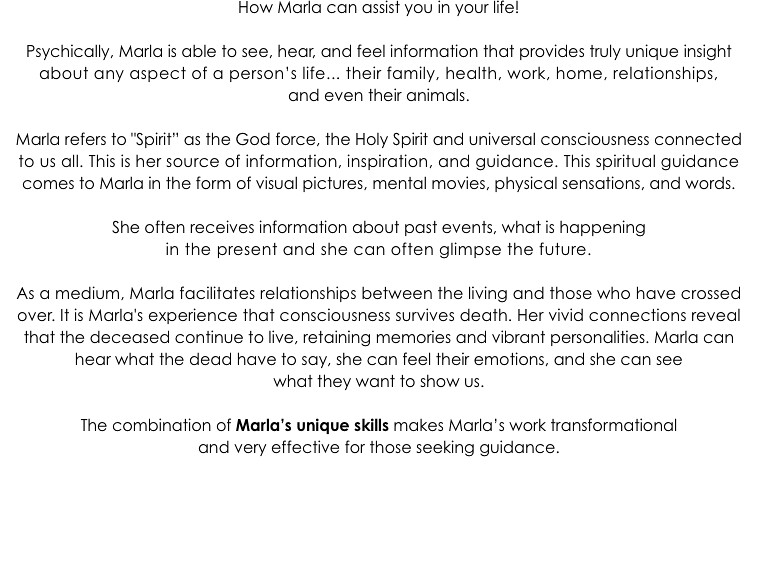The image features a letter on a white background with black text, detailing how Marla can assist you in your life. Emphasized in bold in the concluding paragraph, it explains Marla's unique skills. Psychically, Marla is able to see, hear, and feel information, providing truly unique insights into any aspect of a person's life, including family, health, work, home, relationships, and even their animals. She refers to Spirit as the God Force, the Holy Spirit, and Universal Consciousness, which she identifies as her source of information, inspiration, and guidance. This spiritual guidance appears to her in the form of visual pictures, mental movies, physical sensations, and words. Marla often receives information about past events, current happenings, and can occasionally glimpse the future. As a medium, Marla facilitates relationships between the living and those who have crossed over, using her ability to hear, see, and feel the deceased, who retain their memories and vibrant personalities. Marla's experience asserts that consciousness survives death, making her work not only transformational but very effective for those seeking guidance.